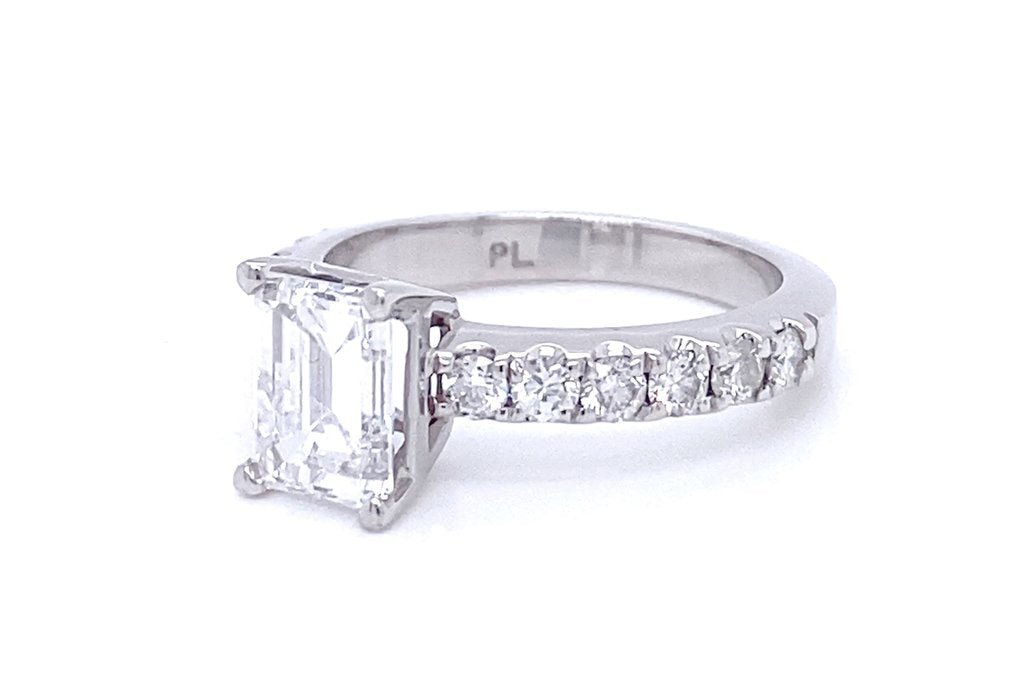This image is a close-up photograph of an elegant engagement ring placed on a white background, revealing a slight shadow. The ring is primarily composed of platinum, as indicated by the "PL" engraving on the inside of the band, giving it a reflective, silver appearance. The band itself is relatively thick and sturdy, transitioning from a flat surface at the top to beveled sides that lead to another flat surface along the edges. 

At the center of the ring, there's a prominent, square-shaped diamond, secured by four protective prongs. This main diamond, cut in an emerald style, is large and flat, giving it significant surface area and making it a focal point. Surrounding this primary stone on each side of the band are six smaller, round-cut diamonds, each approximately a quarter carat, which sparkle brightly and add to the overall luxurious appearance of the ring. The small diamonds continue halfway around the band, offering an assumption that they symmetrically adorn the unseen side as well.

The detailed craftsmanship of the ring and the quality of the stones suggest this is a high-value engagement ring, likely to be cherished deeply.